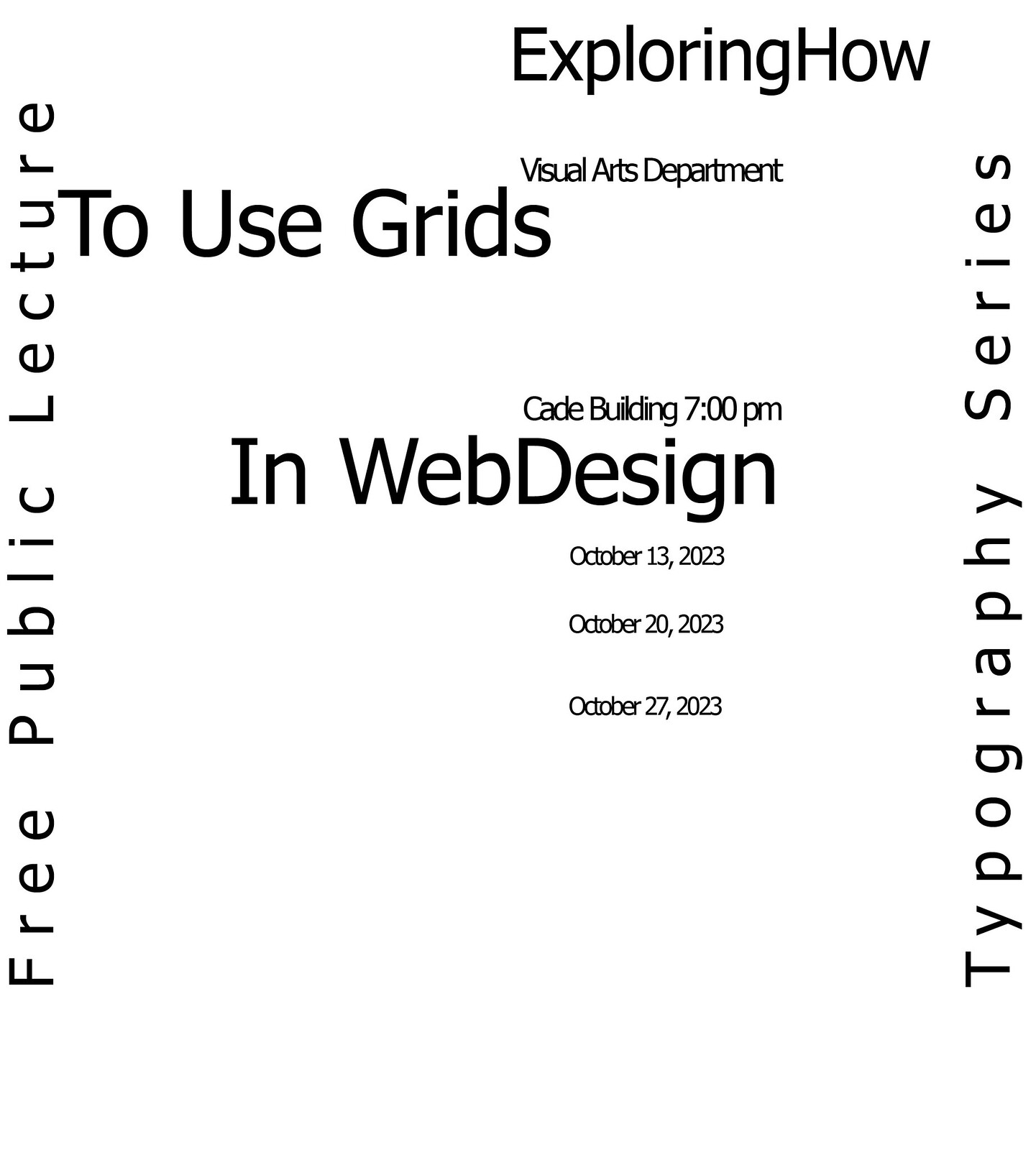The image features black text on a white background, arranged in a visually engaging manner. Along the left border, the text reads "Free Public Lecture" and runs vertically. Similarly, "Typography Series" is written vertically along the right border. At the top center, it states "Exploring How." Directly beneath this, in small text, it says "Visual Arts Department." Below that, in large bold letters, is the phrase "To Use Grids." Following this, in small text are the words "Cade Building, 7 p.m." directly underneath, and then in large bold letters, "In Web Design." At the bottom right of the image, three dates are listed in a column: "October 13, 2023," "October 20, 2023," and "October 27, 2023." The alignment and variation in text size emphasize different elements of the information, enhancing its visual appeal.